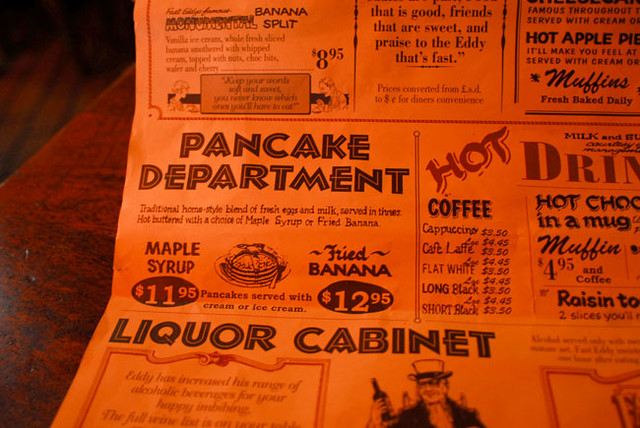In the image, a restaurant or diner menu is shown in dim lighting, creating a slight red color cast that appears to be an artifact of the photograph rather than the menu’s actual color scheme. The menu is designed as a large trifold poster, folded vertically into thirds. Presented on a wooden table, the menu features a somewhat chaotic arrangement, with various font styles and sizes predominately in black text but accented with some red print.

At the top, there's a section titled "Pancake Department." It describes "Traditional home-style blend of fresh eggs and milk served in threes," available either with hot butter and maple syrup for $11.95 or fried banana for $12.95. An illustration of pancakes on a plate accompanies this section. Beneath this is an option to have pancakes served with cream or ice cream.

Following that, there is a "Liquor Cabinet" section, noting an expanded range of alcoholic beverages for patrons' enjoyment. However, the full wine list is cut off in the image. An illustration of a man wearing a top hat holding a bottle adds a whimsical touch to this section.

Further down, there's a partially visible section labeled "Hot Drinks" (abbreviated as "Hot Drin" in the photo), listing options such as coffee, cappuccino, cafe latte, flat white, long black, and short black. Adjacent to these, there is a mention of raisin toast—two slices, though the remainder is obscured. Additionally, a menu item of a muffin with coffee priced at $4.95 and hot chocolate served in a mug is noted.

Overall, the dim lighting and color distortion in the photo make it challenging to discern finer details, but the essential elements of the varied menu offerings are apparent.